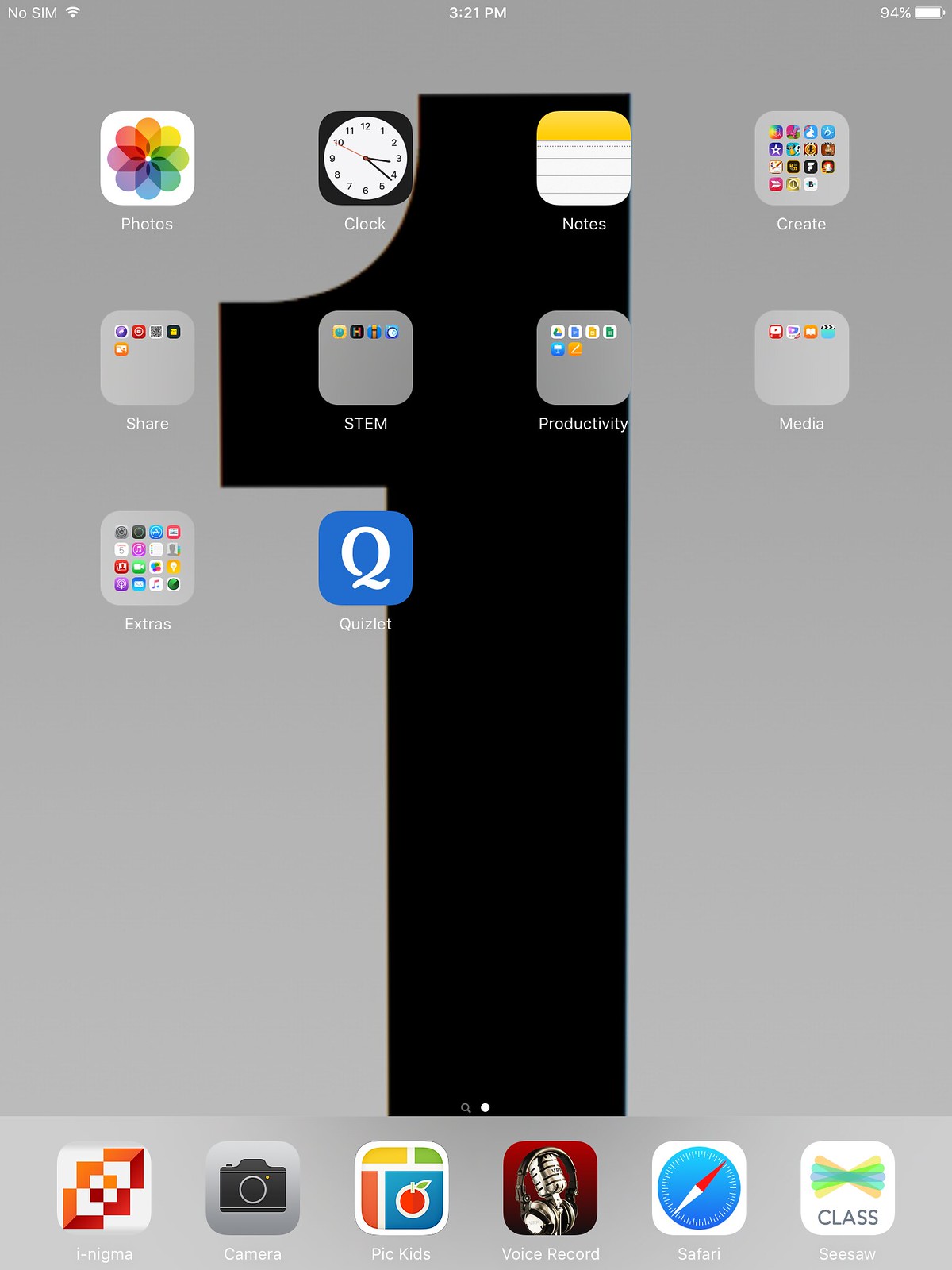The image displays a screen capture from a tablet, identifiable by its size and layout. The background features a gray backdrop with a prominent black structure resembling either the number '1' or a tower. The primary focus is on the tablet’s app tray, showing the icons on the current page. There are four app icons per row, with two full rows and a partially filled third row. 

In the first row, from left to right, are the Photos app, the Clock app, the Notes app, and a Create folder containing numerous other apps. The second row consists entirely of folders named Share, STFM, Productivity, and Media, each containing multiple apps. The third row has a folder labeled Extras, filled with various apps, and an app called Quizlet, characterized by its blue background and a 'Q' logo.

At the bottom of the screen, a fixed bar displays six customized apps: Enigma, Camera, PicKids, VoiceRecord, Safari, and Seesaw.